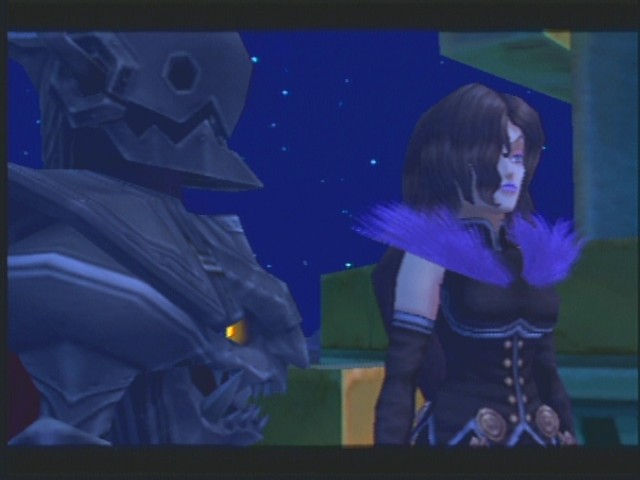The image is a digital illustration set in a night-time scene with a sky rendered in muted blues and greens, speckled with white stars. The background reveals concrete blocks that evoke buildings. On the right side, there is a woman dressed in an extravagant military-style outfit with black cloth, a corset-like top, and long sleeve coverings. Her attire is accentuated by dramatic purple feathers that extend from her chest over her shoulders. She has brown hair, purple eyes, and matching purple lipstick, with arched eyebrows giving her a slightly villainous look. On the left side, facing towards her, is a robotic creature constructed entirely of grey metal with sharp, angular protrusions. This robot features a light emanating from where its heart would be, indicating a sense of life or energy. The overall aesthetic recalls an older fantasy RPG video game, similar in style to early Final Fantasy titles, but with less polished graphics.